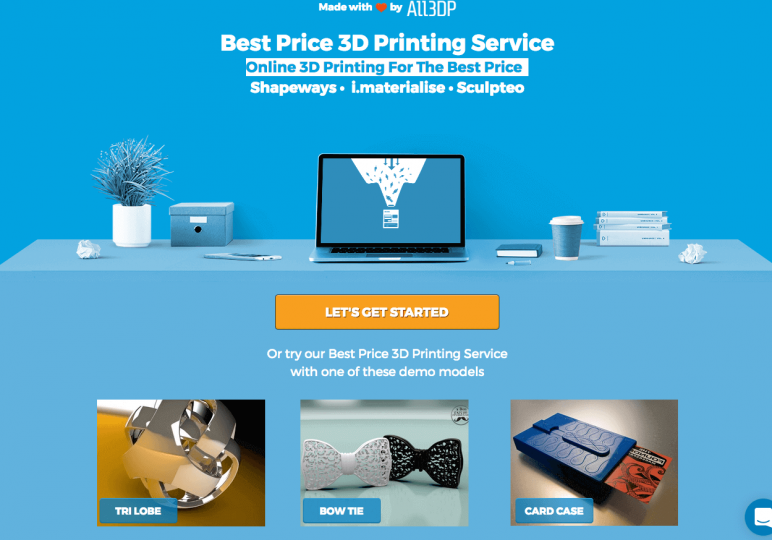This advertisement presents a strikingly monochrome visual in shades of blue and white, creating a minimalist and modern aesthetic. The backdrop features a blue surface adorned with everyday items that include a few plants, a stack of books, a decorative box, wadded up paper, a cell phone, a notebook, a paper coffee cup, and an open laptop displaying its screen. All elements are bathed in a blue-white-black palette, contributing to the cohesive theme.

Centered prominently on the image, the text "Made with ❤️ by AllPrint3DP" stands out, promoting "Best Price 3D Printing Service." The advertisement invites viewers to experience online 3D printing at competitive rates by comparing services offered by Shapeways, i.materialize, and Sculptio. An eye-catching orange button labeled "Let's Get Started" encourages immediate action.

Beneath this call to action, additional text invites users to "try our best price 3D printing service with one of these demo models." Accompanying this invitation are small, detailed images of various 3D-printed items: a trilobe, a bow tie, and a card case. The bow tie and card case showcase intricate design work, while the trilobe appears as interlocking metallic pieces. These example photos illustrate the range and quality of products available through AllPrint3DP’s service, highlighting the precision and creativity achievable by users.

Overall, this advertisement effectively communicates the service's offerings, emphasizing affordability and quality in the realm of 3D printing.